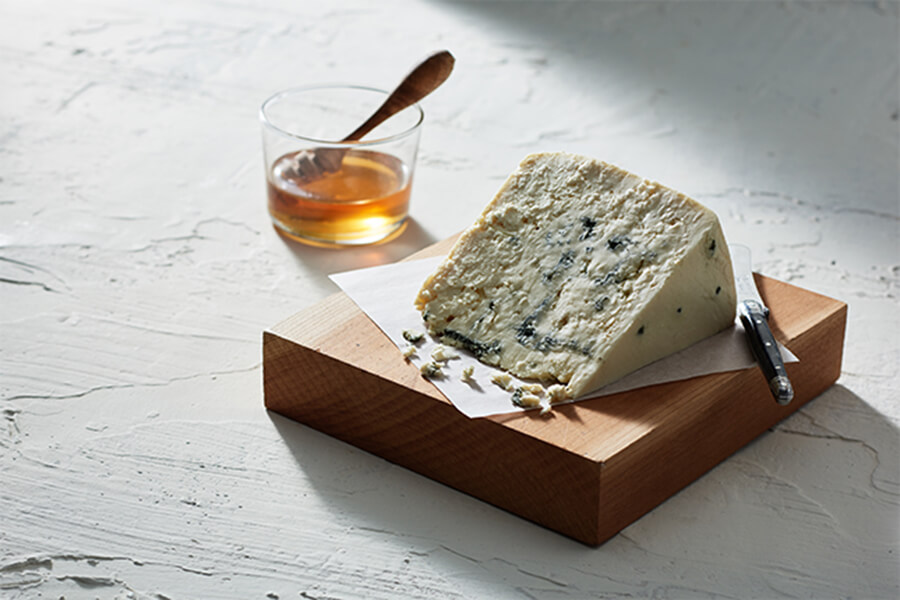The image portrays a large wedge of blue cheese prominently displayed on a piece of parchment paper atop a thick, square wooden block set on a white countertop. The blue cheese, characterized by visible bluish mold marbling throughout and some crumbling onto the paper beneath it, is accompanied by a cheese knife placed nearby. To the right of the cheese wedge, a shot-sized glass half-filled with golden honey sits in the background, catching natural sunlight pouring in from the left. Submerged halfway into the honey is a wooden honey dipper, adding to the rustic and natural aesthetic of the setting. The overall composition captures a warm, inviting atmosphere, highlighting the textures and colors of the cheese and honey against the clean white surface and muddied wooden block.